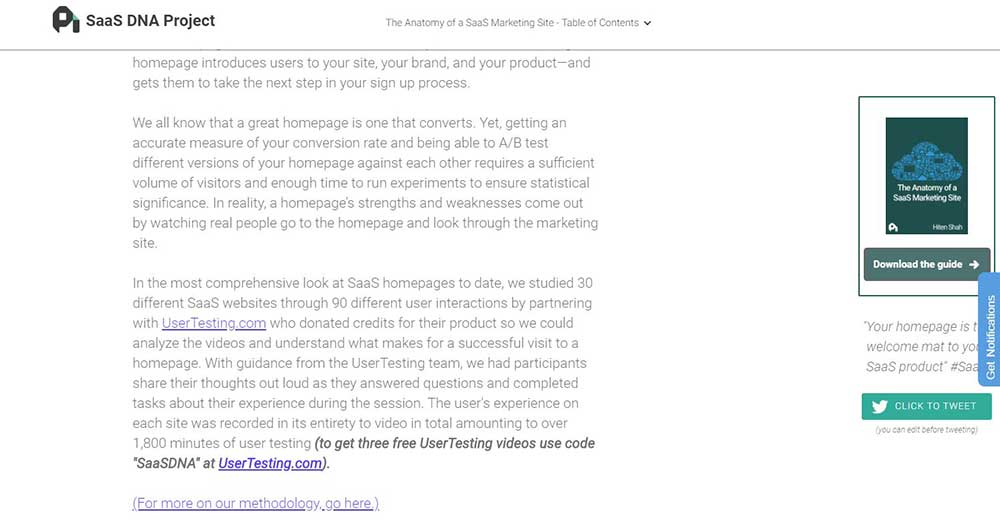This image, sourced from a website, features a predominantly white background. In the upper left corner, there's an icon resembling a black letter "P" with a small green bar extending diagonally towards the bottom right for about a quarter of an inch. Approximately an inch beneath this, a vertical black line descends. Adjacent to this icon, black text in a mix of capitals and lowercase letters reads: "SaasantDNA project". 

Centrally positioned on the page, in small gray lettering, is the title "The Autonomy of SAAS Marketing Site - Table of Contents" accompanied by a dropdown arrow. Below this header lies a gray border that spans the page. Underneath the "DNA" segment in the text, the border continues, followed by text arranged in regular lines consisting of two lines with a space, six consecutive lines, a seventh shorter line, and another small space filled with about ten and a half lines of information. Within these lines, quotations read, "For more on our methodology, go here," underlined and in black font.

On the right side of the image, there is a rectangular box, bordered in blue with a teal interior resembling a cloudy sky with a white overlay. This overlay contains the text, "The Top Anatomy of a SAAS Marketing Site," and includes the same emblem found in the upper left corner. In the bottom right corner of this box, some unreadable text appears. Below, a dark blue tab reads "Download the Guide" in white, next to a right-pointing arrow. Following this, down the right margin, a light blue tab states "Get Notifications" written vertically from bottom to top.

Next to this, additional information is provided in a line, followed by a teal tab featuring the white Twitter bird icon and the phrase "CLICK TO TWEET" in all capital letters.